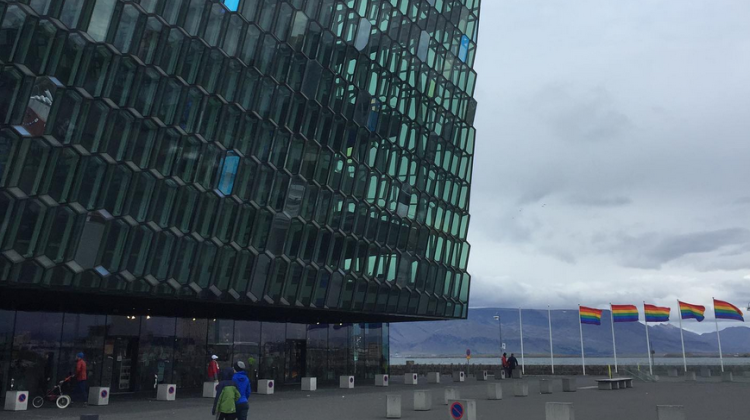This photograph captures a large, tall building with a striking metal and glass facade, predominantly featuring green and gray glass, interspersed with blue and white panels. The architectural design, showcasing numerous rectangular windows across at least 11 stories, exudes an artistic and modern aesthetic. The ground floor is recessed slightly and lined with wide glass windows, adding to its imposing stature. In front of the building, seven flagpoles are prominently displayed, five of which proudly wield rainbow flags that flutter in the wind. A protective row of cement barriers lines the perimeter, hinting at security measures typically seen around significant buildings like museums or public institutions. Scattered around the foreground, a few individuals dressed in colorful and neutral tones mill about, with one person noting a bicycle nearby. The atmospheric backdrop consists of a dreary, gray, cloud-filled sky, contrasting with distant mountains and a body of water, possibly suggesting a scenic yet urban locale.